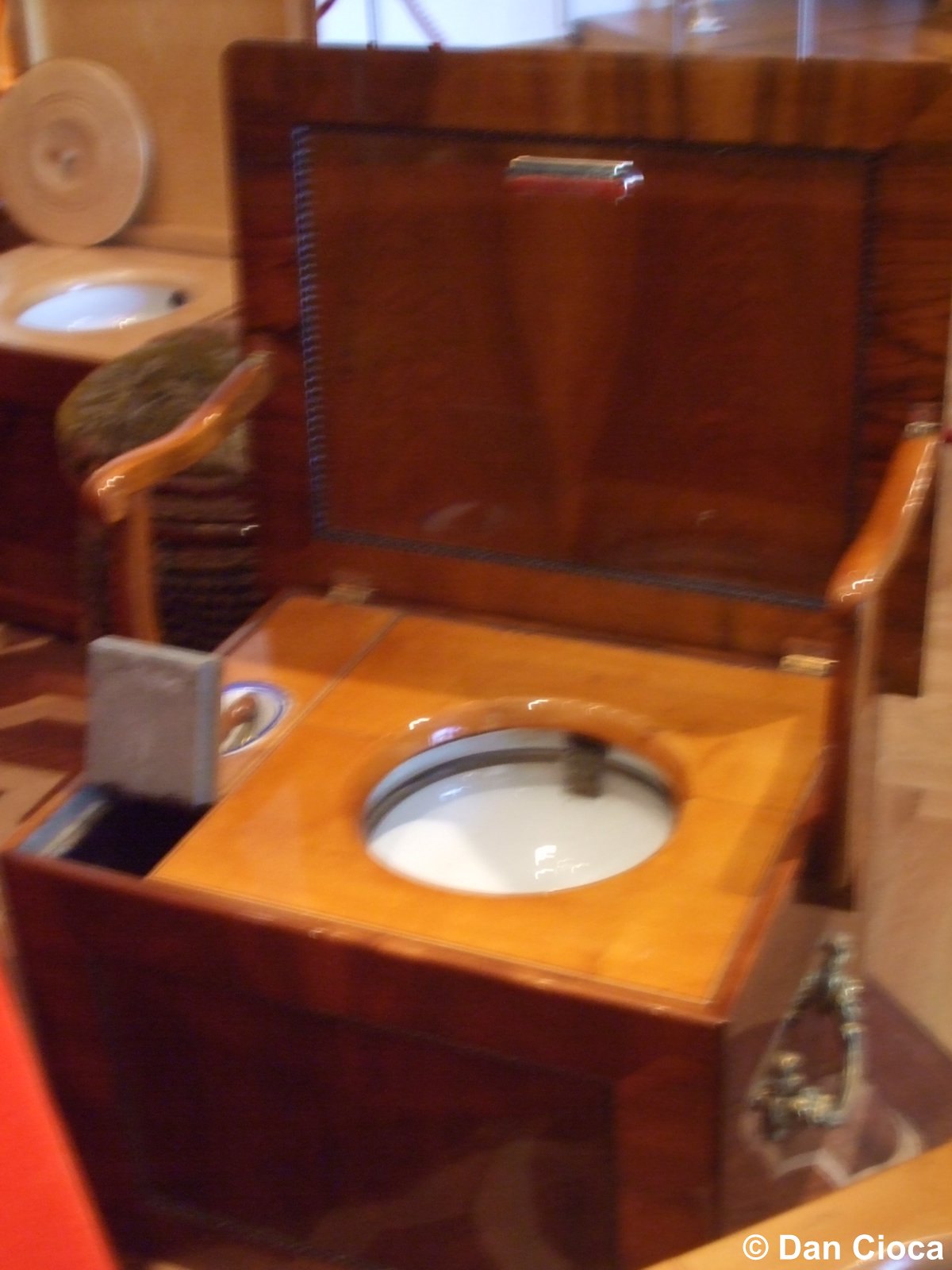This full-color, slightly blurry indoor photograph captures a unique wooden chair that doubles as a toilet, prominently positioned in the center of the image, which is taken on a tiled floor. The chair is made from shiny maple wood and features wooden arms and a square backrest, giving it the appearance of a piece of furniture. The seat of the chair has a circular opening through which a white, concave bowl is visible, rimmed in black. The seat itself is wider than usual, accommodating an additional panel that opens up with a small door. The setting appears well-lit, indicating daytime, possibly in a furniture store or an exhibition. In the background, a window allows some natural light to filter through, and a white, round object is also partially visible. The photograph is copyrighted to Dan Ciocca, with his name noted in the lower right-hand corner. The overall color palette includes shades of red, brown, light brown, gold, white, tan, and gray.